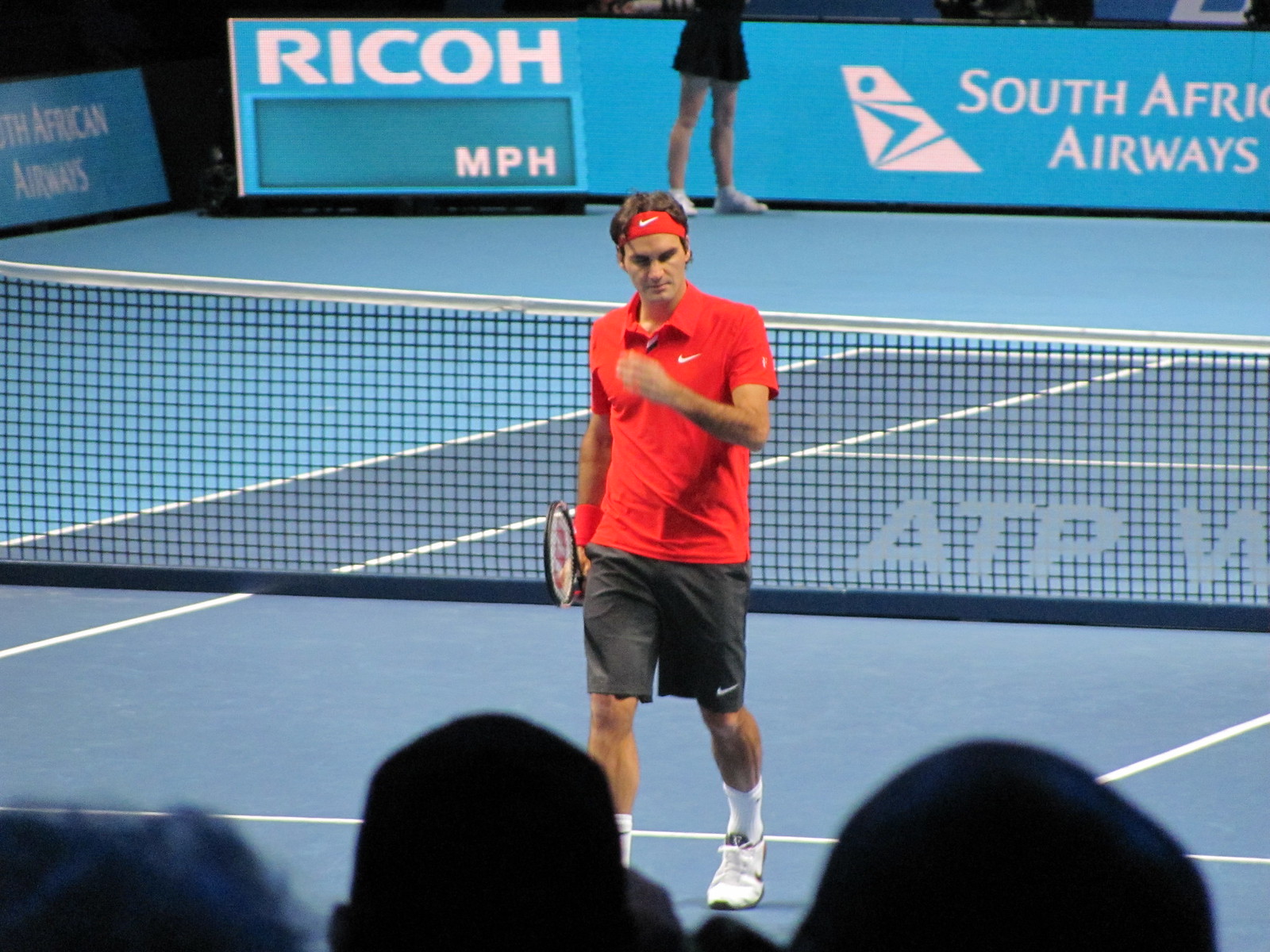The image captures a moment from a professional tennis tournament held on a blue tennis court with white lines. In the foreground, the silhouettes of spectators’ heads can be seen, adding a sense of immersion. The focal point is a male tennis player, appearing to be around 29-30 years old, standing near the net, which has a white striped top and the branding ATPV on it. He is dressed in a red short-sleeved collared shirt, grey shorts, white socks, and white shoes, all of which feature the white Nike Swoosh logo. A red headband with the same Nike logo adorns his forehead. He clutches a Wilson tennis racket in his right hand, identifiable by the red "W" on its strings. Behind him, partially visible, is a ball girl and signage for sponsors like RICOH and South African Airways. The surrounding courts are a lighter shade of blue, enhancing the vibrant sporting atmosphere.